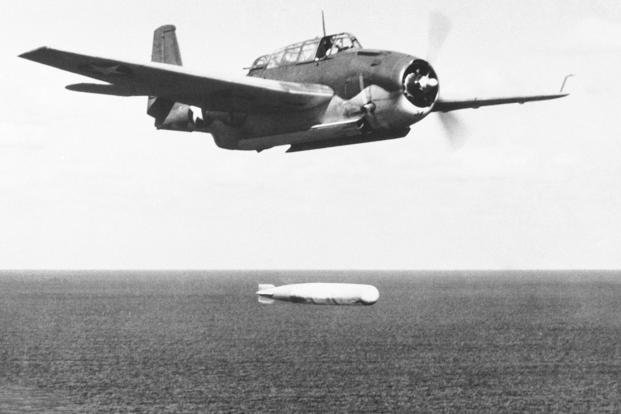This black and white photograph captures a World War II-era Avenger torpedo bomber in mid-flight over a calm ocean. The plane, decorated in its wartime camouflage with a darker upper portion and lighter lower portion, is shown in a three-quarter view from the right side, with the engine running and the canopy open for the pilot. A prominent dark circle with a white star is visible on the left wing and near the tail of the aircraft. Below the plane, suspended in midair, is a long white torpedo that has just been released. The torpedo has not yet hit the water, which occupies the lower third of the image, while the sky fills the upper part. The photograph captures a moment of action during a mission, with the plane appearing to fly level and steady amidst its operation.